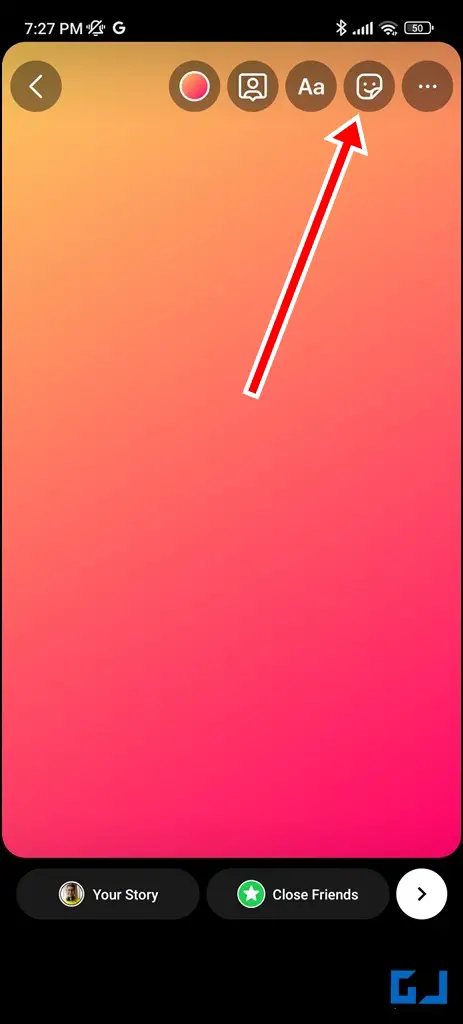A vertically-oriented screenshot taken from a mobile phone, clearly indicated by its long rectangular shape and the presence of typical mobile controls. At the top, there's a thin, black status bar displaying the time (7:27 PM), a "no ring" icon (represented by a crossed-out bell), and the capital letter "G" for Google. To the right, the status bar shows a Bluetooth icon, Wi-Fi signal bars, and a battery level at 50%.

The screenshot appears to be from an Instagram Reel, identifiable because it features the user's profile picture, an option for "Your Story," "Close Friends," and a send button represented by a white arrow at the bottom. The background of the screen is aesthetically pleasing, with a gradient of pink, orange, and yellow hues. Notably, there are no typical app icons visible on the home screen.

A large red arrow points to a smiley face icon among various other icons, suggesting the screenshot is likely part of an instructional guide. However, there is no accompanying description to fully clarify the context. At the very bottom of the screen, there's a "G" and a character resembling a backwards "L," whose purpose remains unclear.